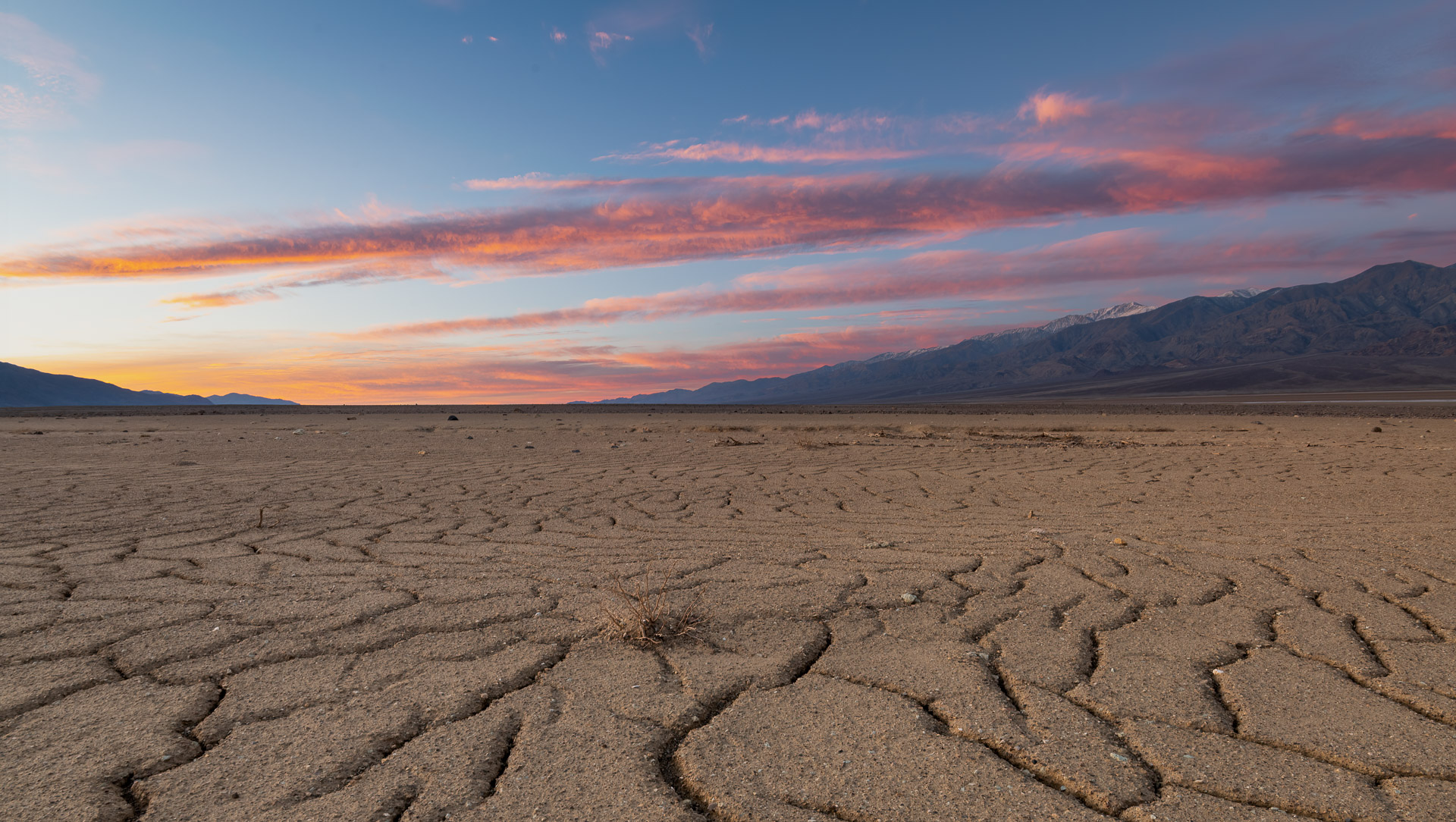The image captures a desolate, cracked desert landscape under the dramatic hues of a setting sun. The foreground consists of dry, brown flatland, riddled with numerous web-like cracks and scattered small white rocks. A single dried-out shrub stands as a lifeless testament to the harsh conditions. In the backdrop, a modest mountain range spans from left to right, with the peaks on the right appearing taller and possibly snow-capped. The sky is a canvas of orange-red and pink clouds, with remnants of blue slowly succumbing to the encroaching darkness of night. The entire scene exudes a sense of arid stillness and solitude.